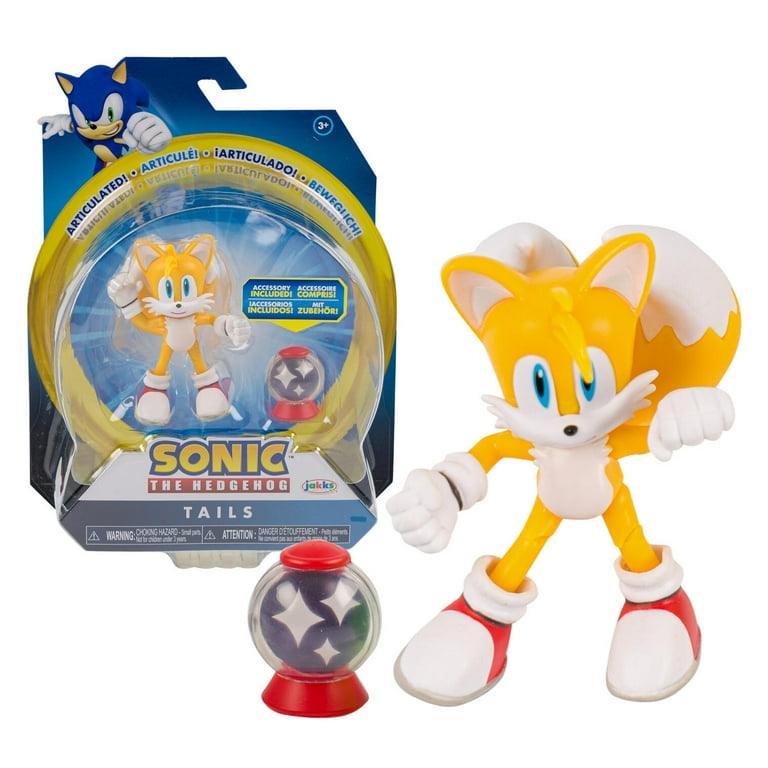This photograph features a detailed scene of a "Sonic the Hedgehog" toy prominently displayed in its original packaging, marketed by the company JAKKS. The toy character, named Tails, is a yellow fox with distinctive attributes including two white-tipped tails, white ears, a white chest, and large blue eyes. Tails is depicted with white gloves, red and white shoes that resemble thick boots, and a white mustache. The packaging is adorned with various elements: 

- In the upper portion, a blue evil-looking cat with yellow ears is present.
- Towards the right, within a white-on-blue circle, there's a label indicating "3+" for the age recommendation.
- The sides of the packaging display multiple translations of the terms "articulated" and "accessory included,” highlighting the toy's movable parts and included extra item.

The cardboard backing behind Tails is predominantly blue, with an image of Sonic in the upper left corner, the signature blue hedgehog character from the franchise. On the packaging, "Sonic the Hedgehog" is prominently displayed under Tails' name.

An accessory resembling a gumball machine is included with the toy, which features a red top and base, a circular glass globe in the middle, and a black section adorned with white diamonds. Near the bottom of the packaging, there are choking hazard warnings.

To the right side of the image, a larger, out-of-package view of Tails showcases the figure's detailed features and articulation points, including movable knees and his two tails. The accessory is also more visible, emphasizing its intricate design.